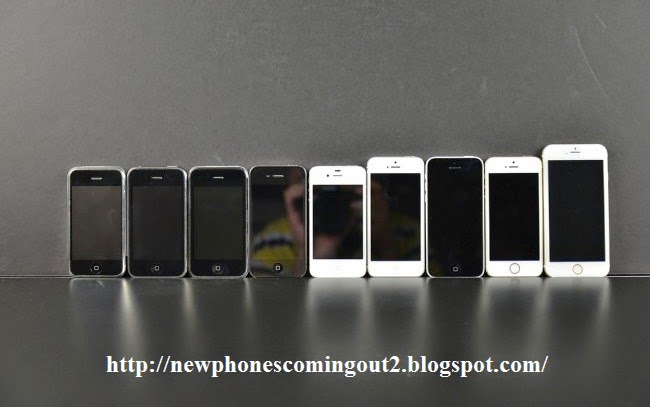The advertisement image showcases nine cell phones lined up from left to right, positioned along the top edge of a shiny, reflective black table against a gray background. The phones increase in size from left to right and display a mix of designs: some with black screens in silver casings, and others featuring white frames. While most screens are off, the fourth phone from the left uniquely reflects an indistinct object. At the bottom of the image, the URL "http://newphonescomingout2.blogspot.com" is prominently displayed, inviting viewers to visit the webpage for more information on the new phones. The photograph composition centers the phones both horizontally and almost vertically, creating a balanced and visually appealing layout.